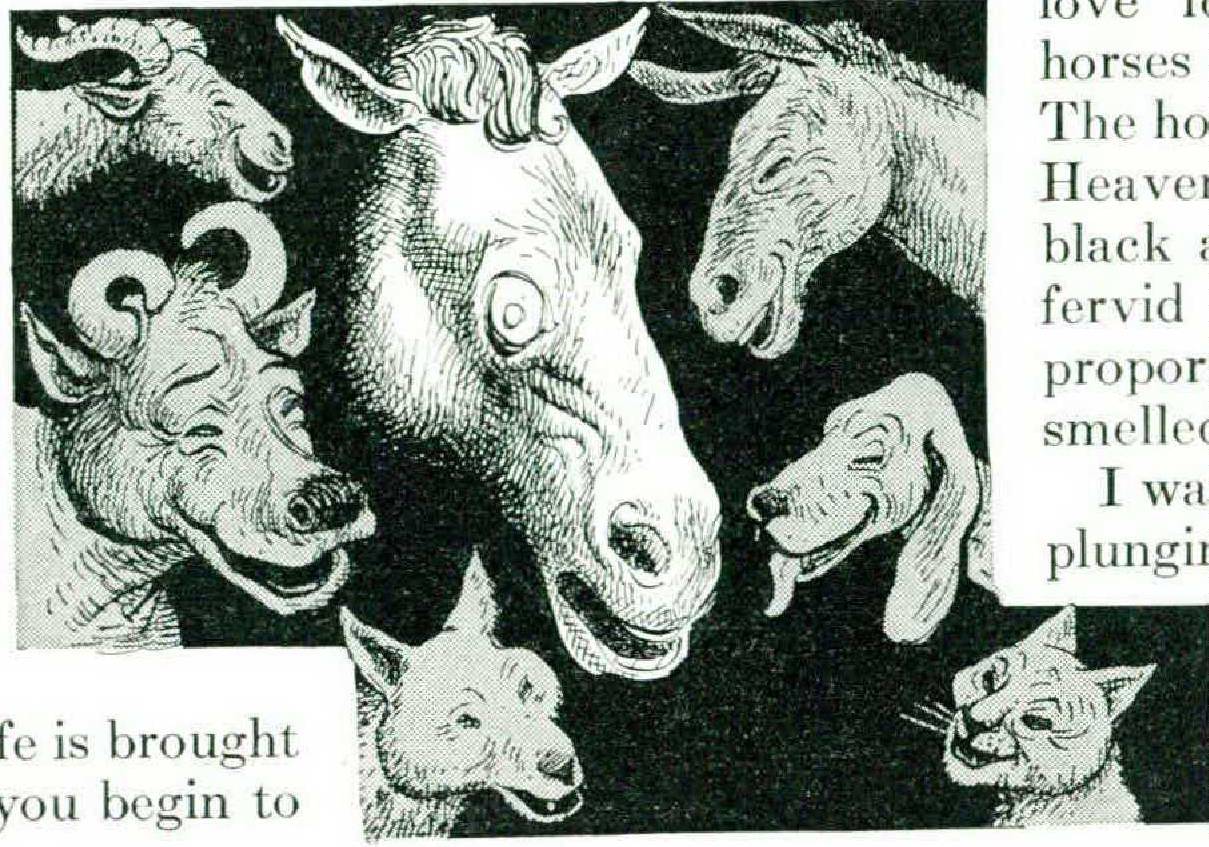This black and white grainy image features a central drawing surrounded by text. The background of the image is predominantly black with white shading, giving it a distinct, high-contrast appearance. In the center of the drawing is the face of a horse, which appears to be scared or nervous. Surrounding the horse are six different animals, all of which are laughing. These animals include:

- Upper left: A goat
- Middle left: A cow
- Lower left: A wolf
- Upper right: Another horse
- Middle right: A dog
- Lower right: A cat

Additionally, a donkey or burrow is also mentioned as one of the animals. 

On the right side of the image, there is a white rectangle containing partially visible text in black, which includes words like "Love, horses, the, H-O, heaven, black, fervid, smelled, I was, plungy." Similarly, in the lower left corner, another text fragment reads "is brought, ye begin."